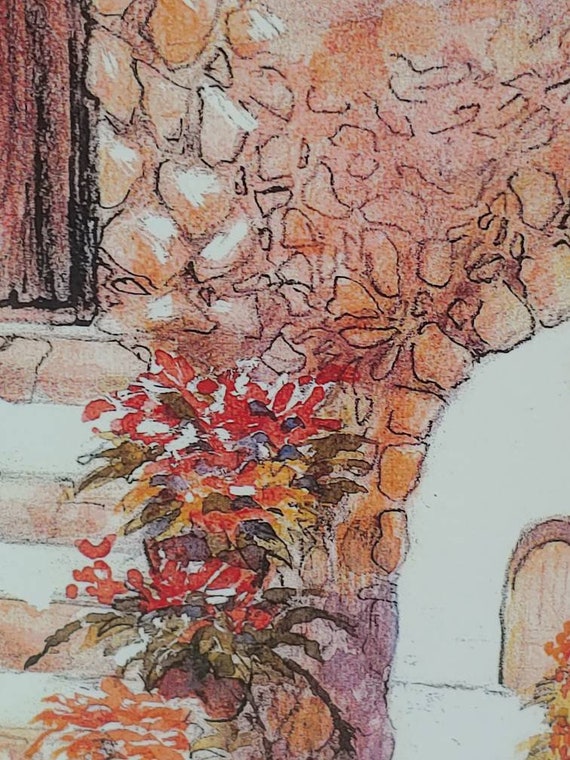The image appears to be a rough hand-drawn depiction of the exterior of an old stone building. The drawing, rendered in black ink with splashes of oranges, yellows, blues, and reds, prominently features a stone archway leading to a walkway. To the left, there's a wooden-framed window above a series of potted plants, which are mainly yellow with hints of red and blue. These plants align along a staircase that ascends towards a door shaded in brown hues. Through the archway on the right side, there's a white wall with another arch-shaped doorway visible in the distance. The scene gives a slightly rough and unfinished impression, likely capturing just a fragment of a larger setting.